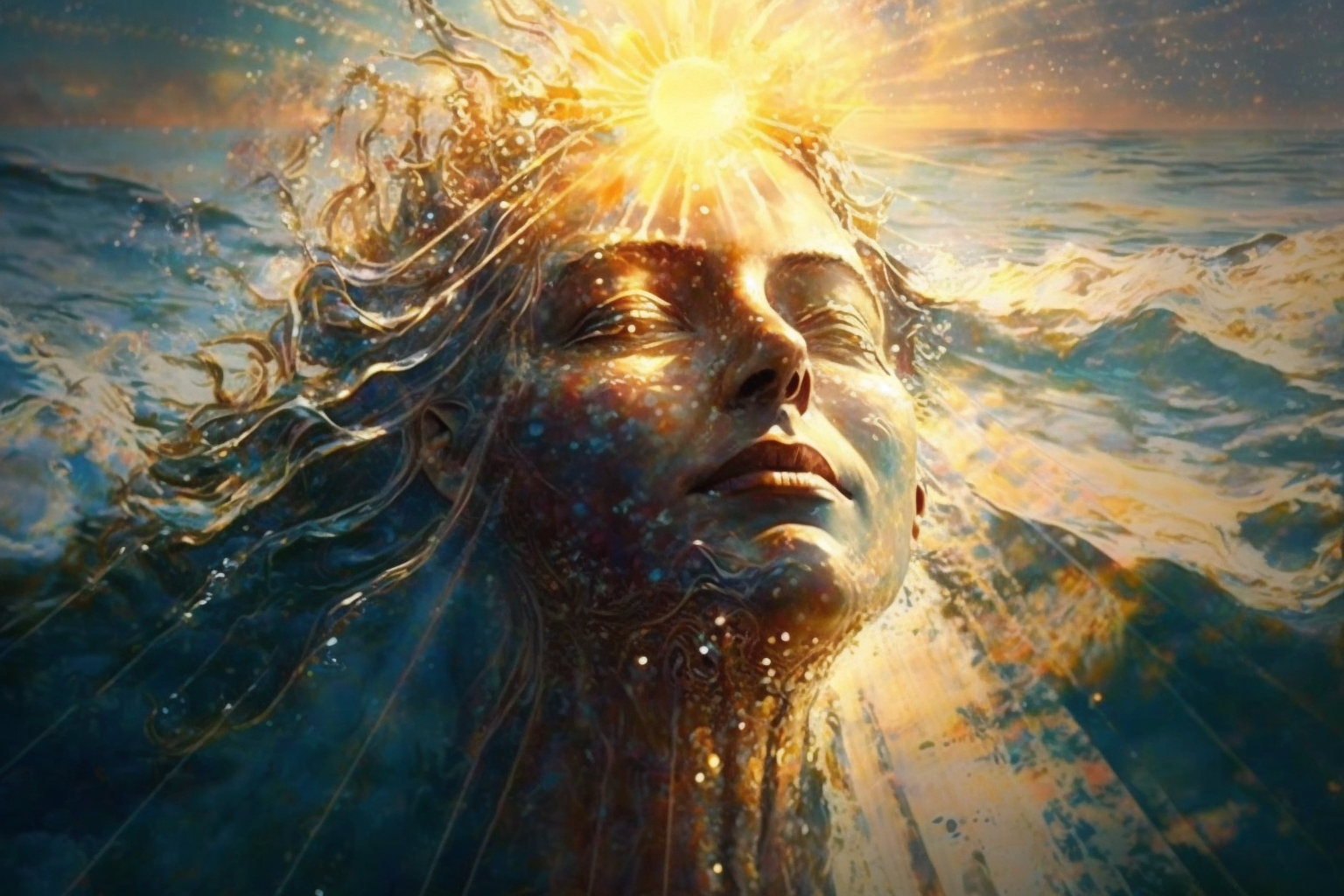The image is a detailed painting, possibly digital art, depicting an ethereal scene where a gigantic woman's head emerges from the rough ocean waves. Her eyes are closed in a serene expression, and her head is tilted slightly upward, almost as if in peaceful contemplation. The forehead of the woman is adorned with a radiant sun, casting brilliant yellow rays that extend across the entire image. Her long, flowing hair merges seamlessly with the turbulent waves, blending shades of blue, white, and hints of gold, suggesting that her hair itself might be made of water. The ocean around her is wild with many white caps, adding to the majestic nature of the scene. The background is an otherworldly sky filled with hues of orange, pink, and blue clouds, perhaps indicating a sunrise or sunset. Her face, decorated with blue dots and painted in a mosaic of blue, white, and yellow tones, seems almost divine. A golden neckpiece is visible, adding to the impression that she might be a goddess. The combination of ocean, sky, and celestial elements evokes a sense of fantasy and grandeur.